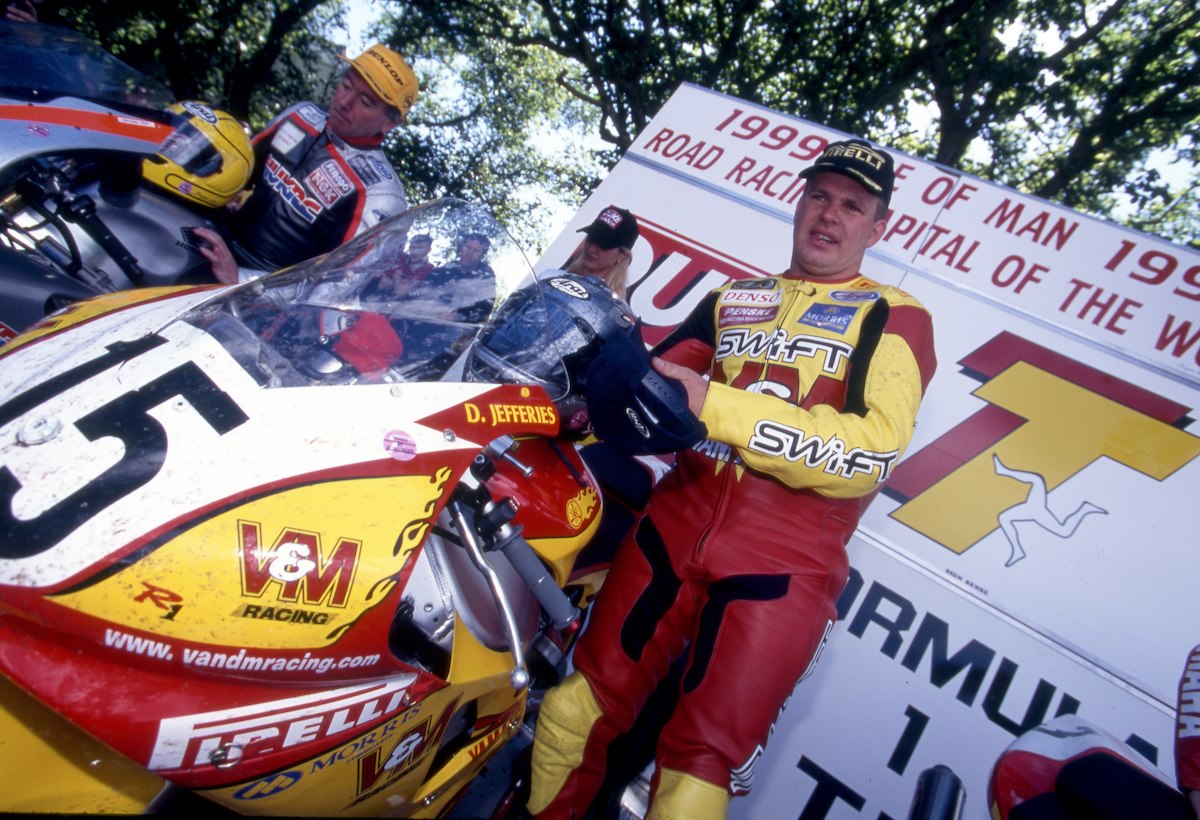This photograph, taken during the 1999 Isle of Man road racing event, captures a candid moment featuring two motorcycle racers, identifiable by the large, partially obscured billboard in the background that reads “1999 Isle of Man, road racing capital of the world.” Both racers are depicted standing beside their motorcycles, having removed their helmets, which now rest on the tanks of their bikes. Each racer wears full racing leathers and a cap, indicating they likely secured top positions in the race.

The primary motorbike, prominently displayed at the center of the image, is adorned in red and yellow colors. The zippered one-piece suit of the racer next to this bike displays the name "D. Jefferies," marking him as a notably recognized participant. His racing suit is red and yellow, matching his bike, and bears the emblem “Swift” in black font outlined in white. To the right of the image, another bike appears, albeit more distantly, in red and silver hues. 

The photograph is taken at a slight angle, directing the subjects' heads towards the top right corner. The distant background reveals a serene blue sky punctuated by green-leaved trees. A large poster features part of the Isle of Man’s well-known triskelion logo – three legs connected together, symbolic of the island’s heritage. Both racers, their motorcycles, and the celebratory ambiance collectively convey the high stakes and exhilaration of this renowned racing event.